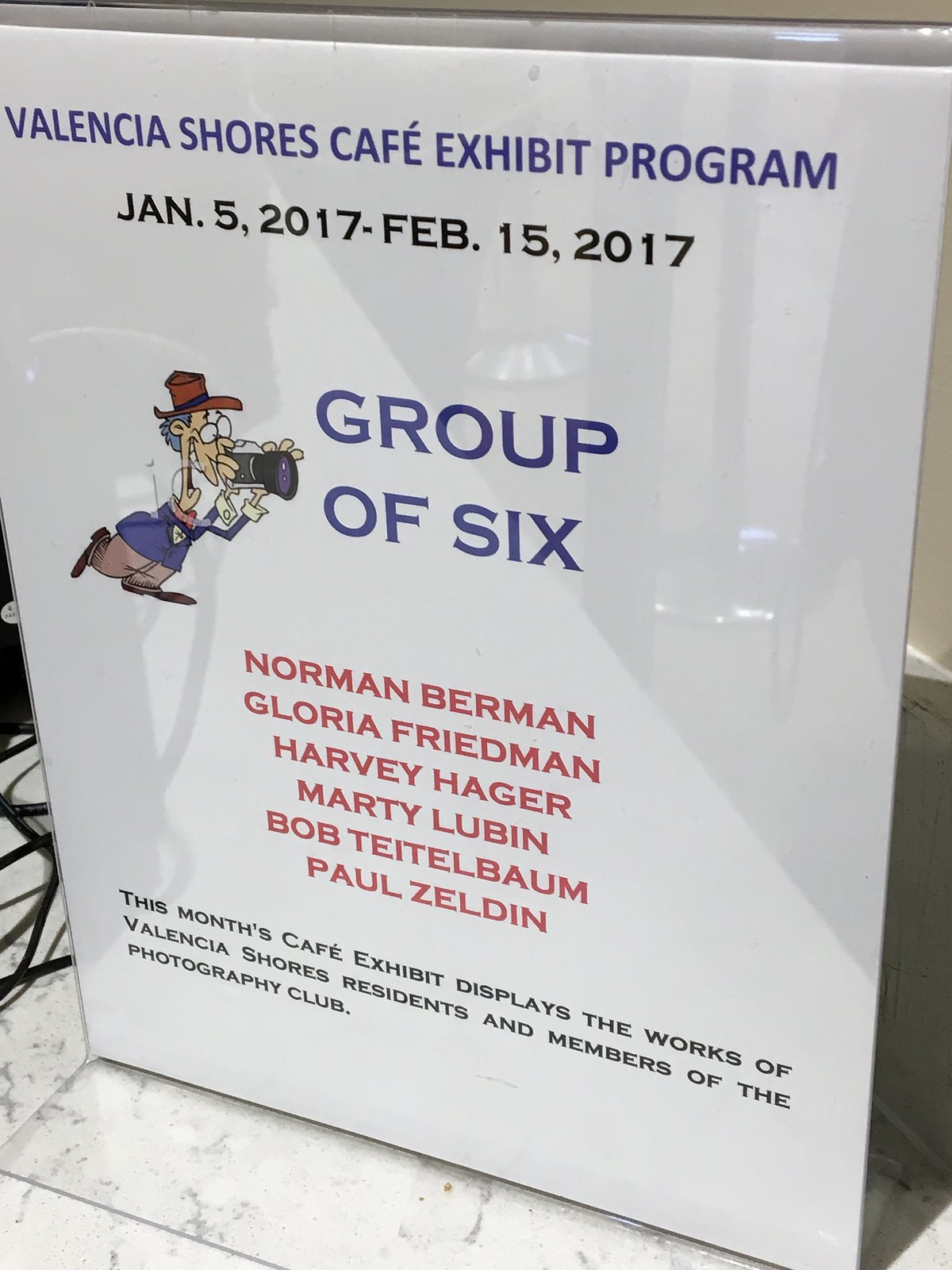The image depicts an indoor scene, featuring a white tiled floor with gray marble-like designs. In the background, a cord or cable is visible. Dominating the frame is a sign placed in an acrylic holder and set on a table. This sign, with a white background, has blue lettering at the top that reads "Valencia Shores Cafe Exhibit Program," and black lettering below indicating the event dates, "January 5, 2017 to February 15, 2017." The sign showcases a cartoon illustration of a man with a hat, camera, purple shirt, and brown pants, actively taking a photograph. Accompanying this illustration, the blue text "Group of Six" is followed by names in red—Norma Bergman, Gloria Friedman, Harvey Hager, Marty Lubin, Bob Teitelbaum, and Paul Zeldin. Additional black text explains, "This month's cafe exhibit displays the works of Valencia Shores residents and members of the Photography Club." The sign promotes a photography exhibit featuring artwork created by members of the Valencia Shores community.